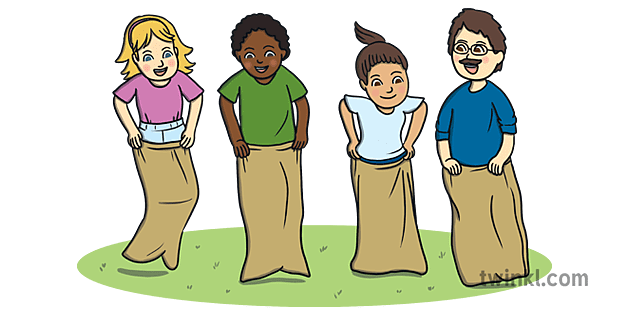The illustrated image, reminiscent of a children's book, captures a lively potato sack race set on vibrant lime green grass. Four characters are animated mid-jump inside tan sacks. On the far left, a young Caucasian girl with blonde hair in a purple (sometimes described as pinkish) shirt and blue jeans energetically participates. To her right is a young African American boy with curly black hair, sporting a green shirt. Next to him is a possibly Hispanic girl with dark brown hair tied in a ponytail, wearing a white shirt. Completing the lineup on the right is an older Caucasian man, perhaps their teacher, distinguished by his glasses, mustache, blue t-shirt, and short hair. The white background of the image is punctuated with the logo "twinkl.com" in the bottom right corner, suggesting digital artwork.